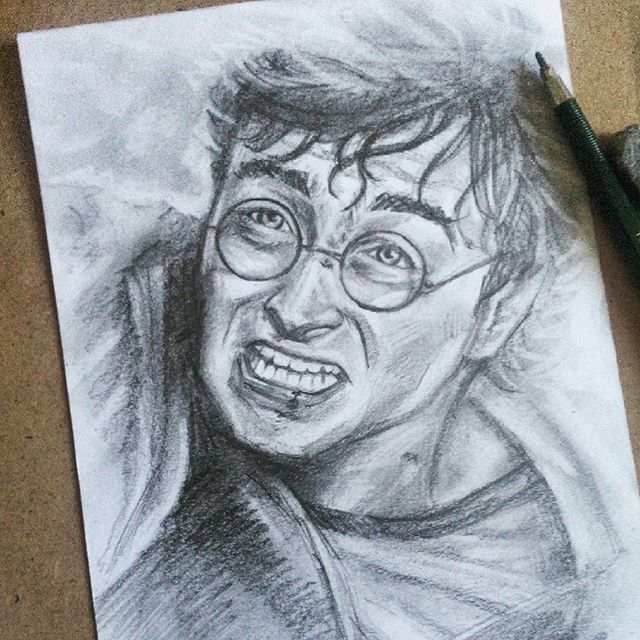A meticulously crafted pencil drawing of Harry Potter is showcased here, pinned at a diagonal angle on a cork board backdrop. The rectangular sheet of drawing paper exhibits a detailed portrayal of Harry Potter's face and torso. The young wizard is depicted with his mouth open and teeth clenched, conveying a sense of intensity or determination. Signature round-framed glasses accentuate his familiar features. Resting atop this captivating artwork is a pencil, suggesting the artist’s tool of creation, adding an authentic touch to the presentation.